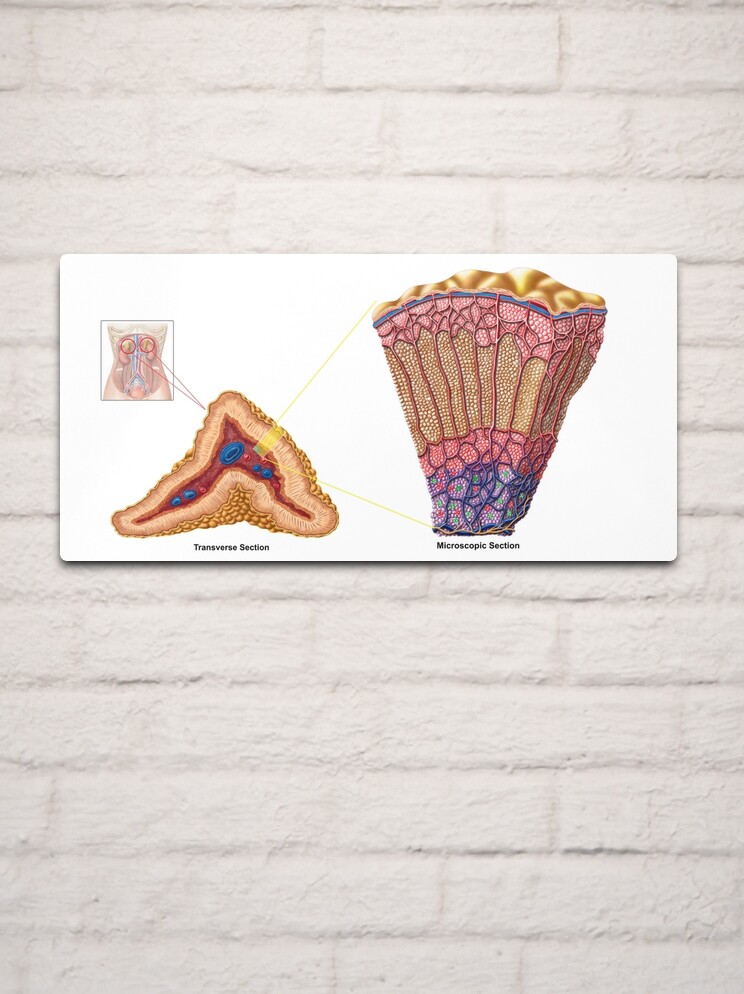The image displays a detailed medical diagram of a human body, focusing on an anatomy segment. The background of the diagram is white, and it is mounted on a white-painted brick wall. On the left-hand side near the top, there's a faded depiction of a human torso with arrows pointing to a specific area, which seems to be in the abdominal region. Adjacent to it, the enlarged view labeled "transverse section" showcases a bumpy area with red, blue, yellow, and brown colors, representing various cells and tissues. Next to this section, there's another zoomed-in view labeled "microscopic section," displaying a smaller segment with intricate details in yellow, pink, orange, and blue. Each section of the diagram is clearly distinguished, providing a comprehensive view of the anatomical and cellular structures.